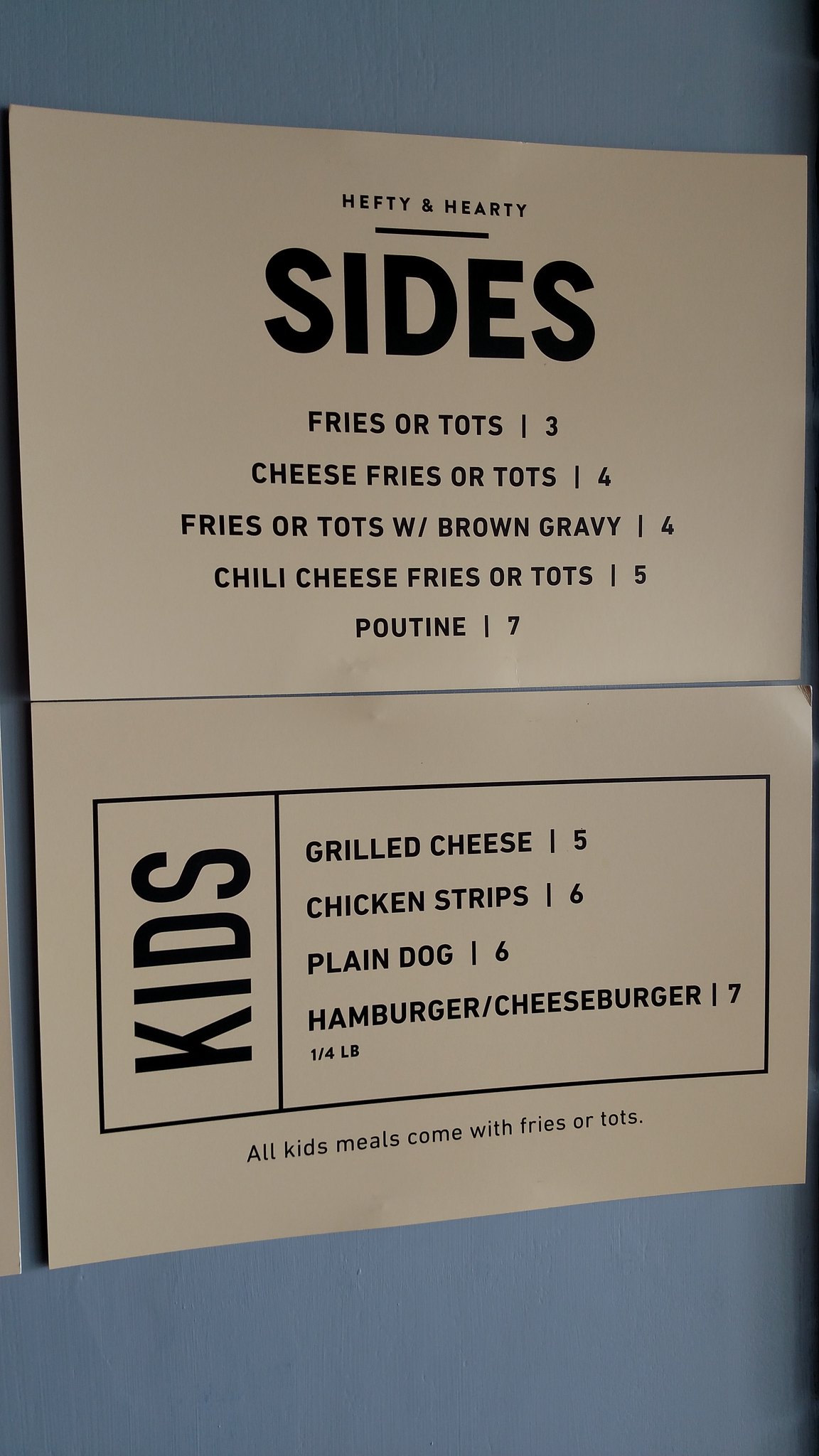The image captures a pair of plain, worn paper signs posted on a desaturated blue wall, possibly inside a dimly lit corner of a restaurant. The top sign, under the heading "Hefty and Hearty Sides," lists various options such as Fries or Tater Tots ($3), Cheese Fries or Tots ($4), Fries or Tots with Brown Gravy ($4), Chili Cheese Fries or Tots ($5), and Poutine ($7). Below, the second sign is labeled "Kids" and specifies that all kids' meals come with Fries or Tots. The kids' meal options include Grilled Cheese ($5), Chicken Strips ($6), Plain Hot Dog ($6), and both Hamburger and Cheeseburger ($7), with the latter described as a quarter-pound patty.

The lighting in the photograph is minimal, likely from a distant window, casting insufficient light to brighten the scene. The paper shows signs of age, appearing yellowed and gray, adding to the overall somber and uninviting atmosphere. Other snippets of paper are barely visible at the edges, indicating additional but unspecified information outside the frame. The focus remains tight on these two menus, with no other noteworthy elements within the image's confines.